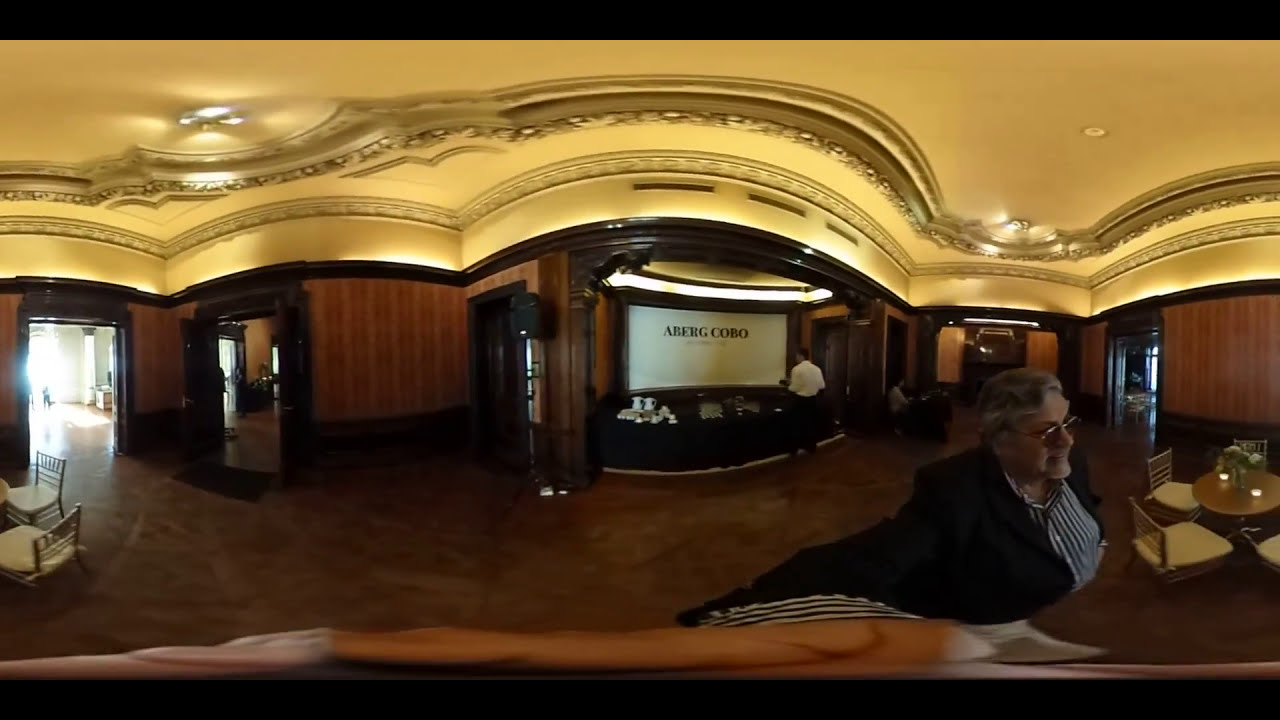In the image, you find yourself inside an ornate, old-timey theater or conference hall brimming with intricate details and a sense of historical charm. Dominating the ceiling, ornate, gold-accented carvings and crown moldings stretch along, forming a lavish three-foot border that adds to the grandeur of the space. The ceiling has a unique design with multiple curves, resembling an undulating wave or bubble pattern. The room showcases luxurious wood paneling and flooring, contributing to its sophisticated ambiance.

Positioned towards the center, you see a long black table adorned with coffee, snacks, and teacups, suggesting a refreshment station. Behind this table stands a man, casually enjoying the treats, wearing a black shirt with a blue and white striped undershirt. This man also appears in the right foreground, distorted due to the 360 panoramic shot – his right arm extended unnaturally towards the ceiling's ornate bubbles.

A large sign with the words "Aberg Kobo" presides over the refreshment table, possibly indicating the name of the company or event. Surrounding the area are several wooden doors with dark frames, hinting at access to other parts of the grand theater. The walls of the room are a rich brown, complementing the stateliness of the scene. Light fixtures above subtly illuminate the space, casting a warm glow over the entire setting. Another man, dressed in business attire and holding a camera, stands before the sign, perhaps capturing the elegance of the surroundings or the moment itself.